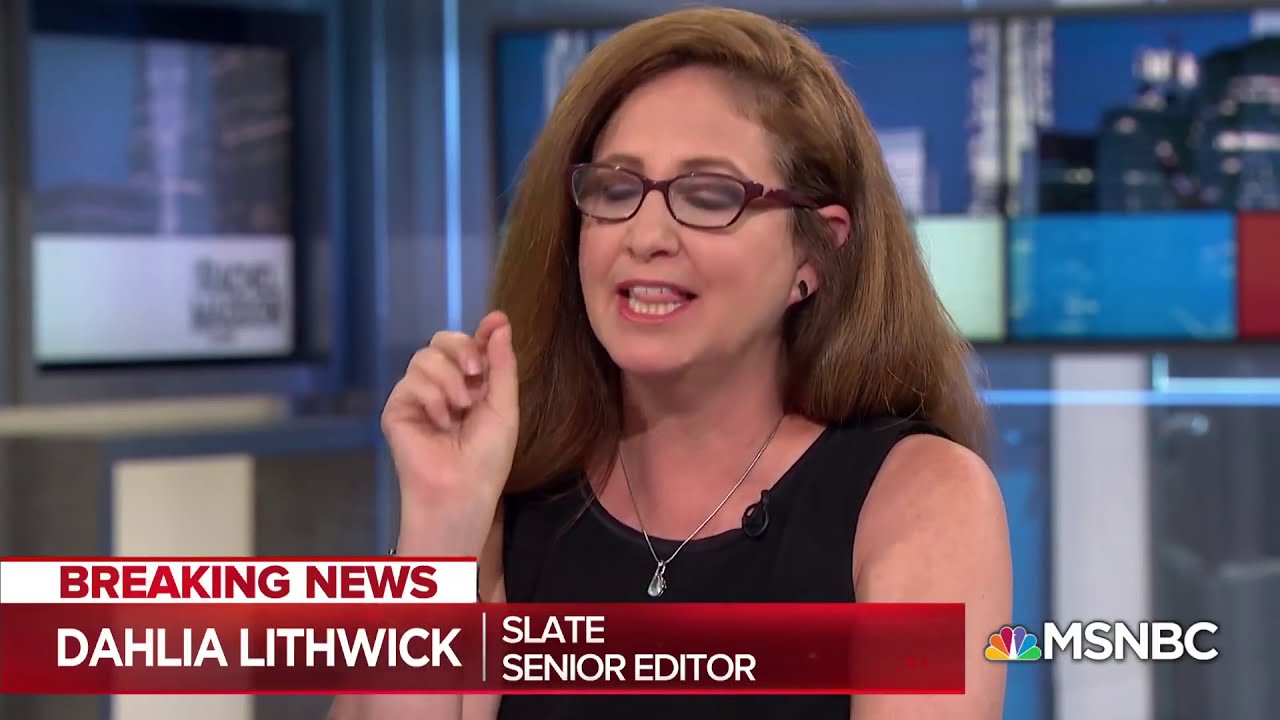The image is a close-up screenshot from a news broadcast on MSNBC, identifiable by the MSNBC logo and peacock icon in the lower right corner. The broadcast features a title in a red rectangle at the bottom left stating, "Breaking News, Dahlia Lithwick, Slate Senior Editor." The main focus is on Dahlia Lithwick, who is speaking mid-sentence with her mouth open, revealing her tongue between her teeth. She is wearing maroon-colored glasses and a black sleeveless top with a microphone clipped to it, along with a silver necklace with a pendant. Her thick, dark brown hair frames her face, and she has one hand raised with her pointer finger and thumb pressed together as she gesticulates. The background features an out-of-focus TV studio setup with colorful elements, windows, and computer screens.